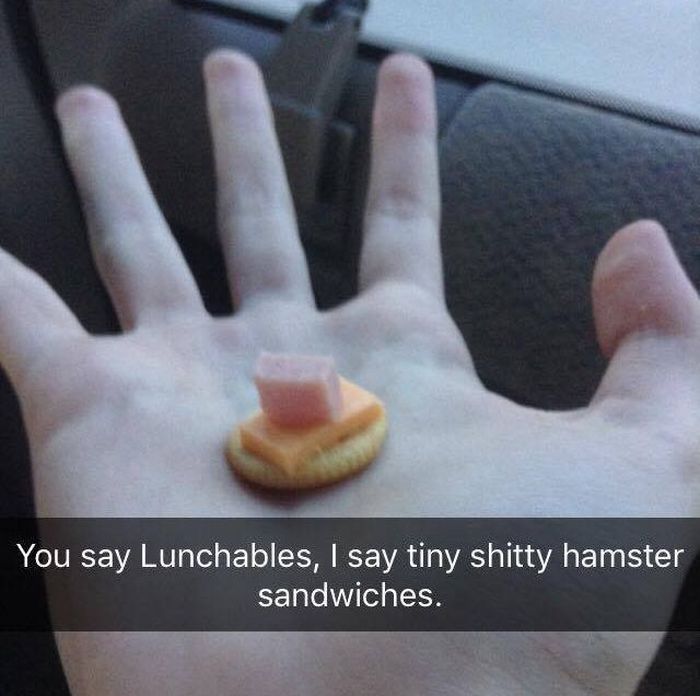The photograph captures a left hand of a Caucasian individual, possibly a teenage or young adult male, held palm-up with fingers spread and thumb slightly bent. Nestled in the center of the palm is a Ritz cracker topped with a square piece of orangish-yellow cheese and a rectangular cube of pink ham. The setting appears to be the interior of a car, evidenced by a fuzzy, diagonally-oriented gray windowsill in the top right corner and a grayish-blue triangular patch that could be the sky peeking through. A gray to black divider is also visible. Overlaying the lower part of the image is a semi-opaque gray banner with white Comic Sans text humorously reading: "you say Lunchables, I say tiny shitty hamster sandwiches." The photograph, bordered by the meme text, suggests it is meant to be amusing and could easily be shared online, particularly as a lighthearted commentary on Lunchables in the United States.